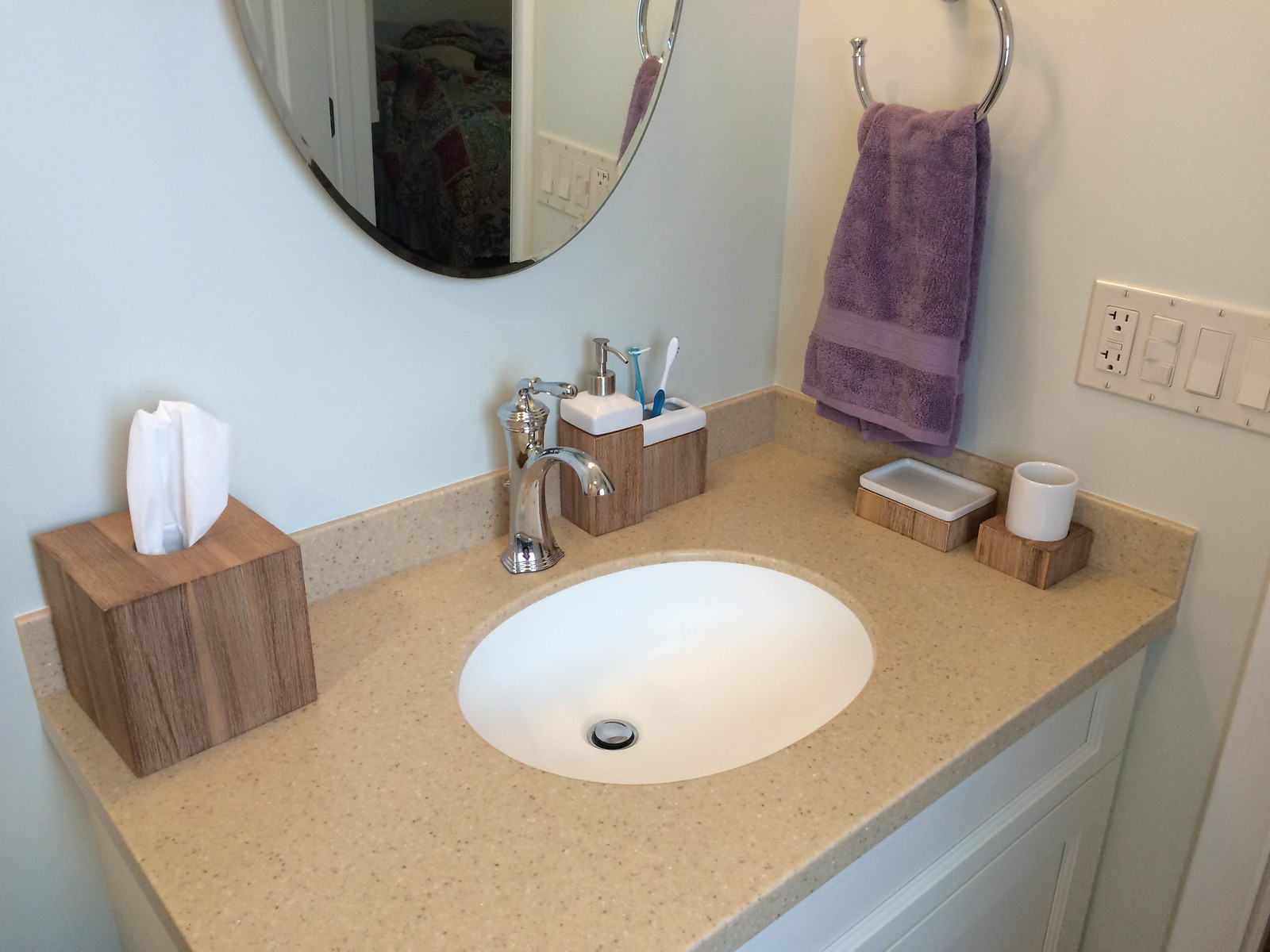The image depicts a bathroom sink photographed from an angular left-hand side perspective, providing a slightly off-centered view. The countertop of the sink is adorned with light brown marble, contributing a touch of elegance to the setting. The lower portion of the image reveals part of the white cabinet beneath the sink.

Above and behind the sink, an oval-shaped mirror occupies the space, capturing a reflection of the room's elements. Within the mirror's reflection, light switches and a portion of a hand towel, which is purple and hangs from a hook, can be seen. The reflection further reveals glimpses of an adjoining bedroom, including a door.

On the left-hand side of the sink, a wooden textured box serves as a tissue holder. Adjacent to the tap, on the right-hand side, sit a soap dispenser and a toothbrush holder, both sharing the same wooden texture and design. Mounted on the wall next to the sink is another purple hand towel, beneath which stands a wooden box container similar to the earlier one. Another wooden container neighboring it holds a glass on top. Above these containers, several light switches are visible, completing the detailed portrayal of this bathroom scene.